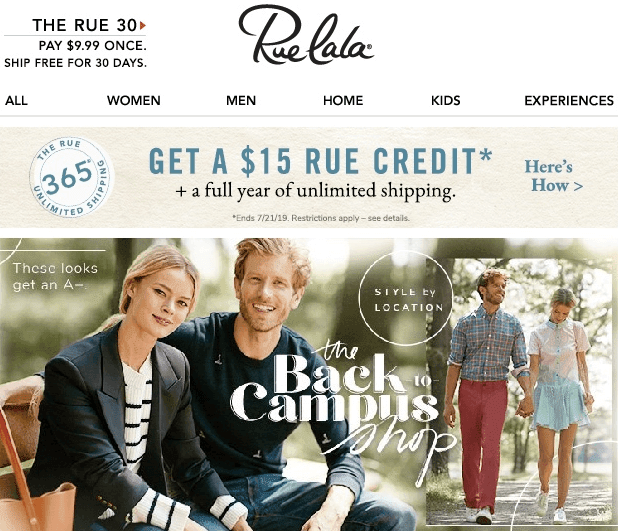Certainly! Here is a cleaned-up, detailed caption for the image:

---

The homepage of the Rue La La (R-U-E L-A L-A) website features a prominent logo centered at the top against a white background, with the name "Rue La La" displayed in an elegant italic font. Directly below the logo, a full-width navigation bar is neatly laid out, listing categories from left to right as follows: Women, Men, Home, Kids, and Experiences.

Taking up much of the page is a banner promoting the "RUE 365 Unlimited Shipping" offer. On the left side of the banner, text reads "Get a $15 RUE Credit" with an adjacent asterisk noting terms applicable from N-7-21-19, advising visitors to see details for restrictions. Below this, the offer promises "A Full Year Unlimited Shipping" in bold black font. To the right, a button labeled "Here's How" invites users to learn more.

Beneath the banner, two images dominate the lower section. On the bottom left, a larger image showcases a man and a woman sitting on a bench dressed in outdoorsy, L.L. Bean-style attire, captioned "These Looks Get an A-." On the right, another section highlights the "Back to Campus Shop," suggesting styles curated by location.

In the top-left corner of the homepage, the "RUE 30" promotion is displayed. Underneath this, a succinct tagline reads "Pay $9.99 Once, Ship for Free, 30 Days," emphasizing the site's shipping deal.

---

This detailed caption provides a comprehensive description of the homepage layout, highlighting each section's key features and placements.